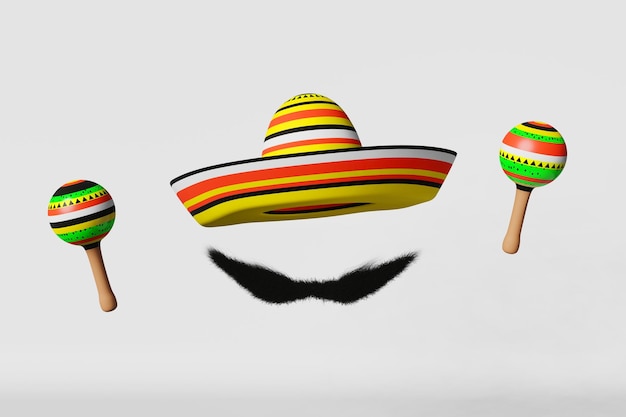In this whimsical and festive image, a traditional Spanish costume appears to float against a soft off-white background, seemingly held up by an invisible figure. At the top, a colorful sombrero hovers where a head would be, adorned with vivid stripes of black, white, dark orange, yellow, green, blues, and reds, creating an eye-catching pattern that radiates from the brim to the crown. Flanking the sombrero, two wooden maracas float in the positions hands would occupy, each decorated with a harmonious mix of green, yellow, black, white, and red, featuring stripes, triangles, and dots. Below the sombrero, an exaggerated, long black mustache hangs in mid-air, so wide it spans the brim of the hat. The mustache is fuzzy and detailed, giving it a playful, almost animated appearance, reminiscent of the magnetic beard toy. This charming ensemble captures the lively spirit of a fiesta, blending traditional elements with a touch of surrealism.